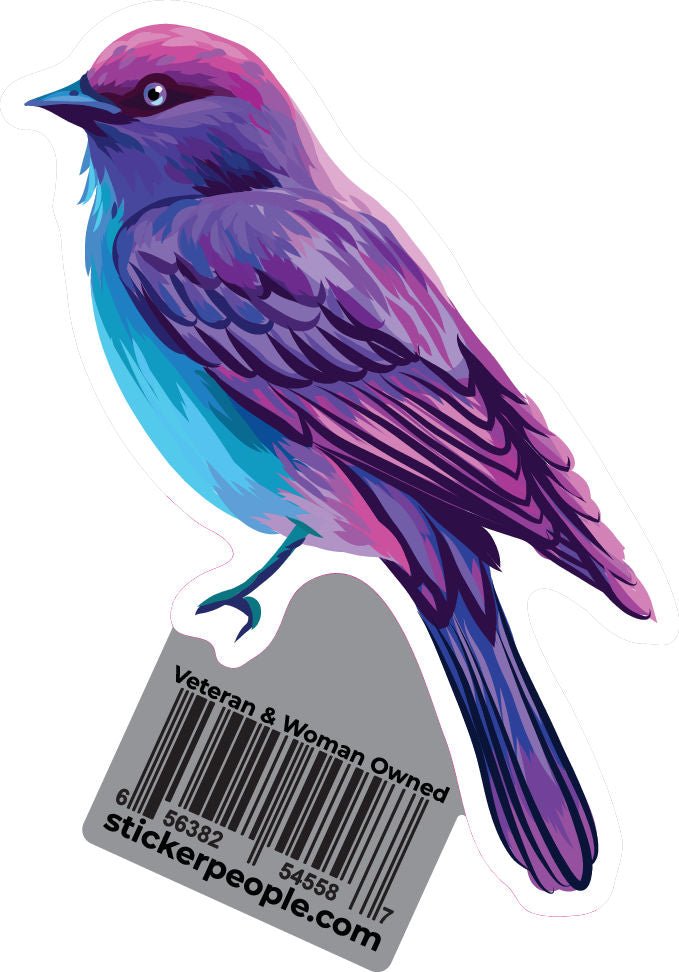This image is a close-up of a vibrant, animated sticker of a bird on a white background. The bird is depicted in a side view, with its head facing the upper-left corner of the image and its tail pointing downwards to the right. The bird features a lively blend of colors: its wing and tail feathers are predominantly purple, bordered with black highlights. The head showcases a mix of dark and light purple, with the top part being a brighter purple shade. The beak is a striking blue, and the underbelly consists of various shades of blue, ranging from a light, neon blue to deeper aqua tones. The bird's foot is also blue. Outlined in a very light gray, the bird stands out vividly against the white background. Below the bird, there's a gray sticker with black text stating 'Veteran and Woman Owned.' Beneath this text, there's a black barcode with the number '656382545587' and the website 'StickerPeople.com' written underneath.